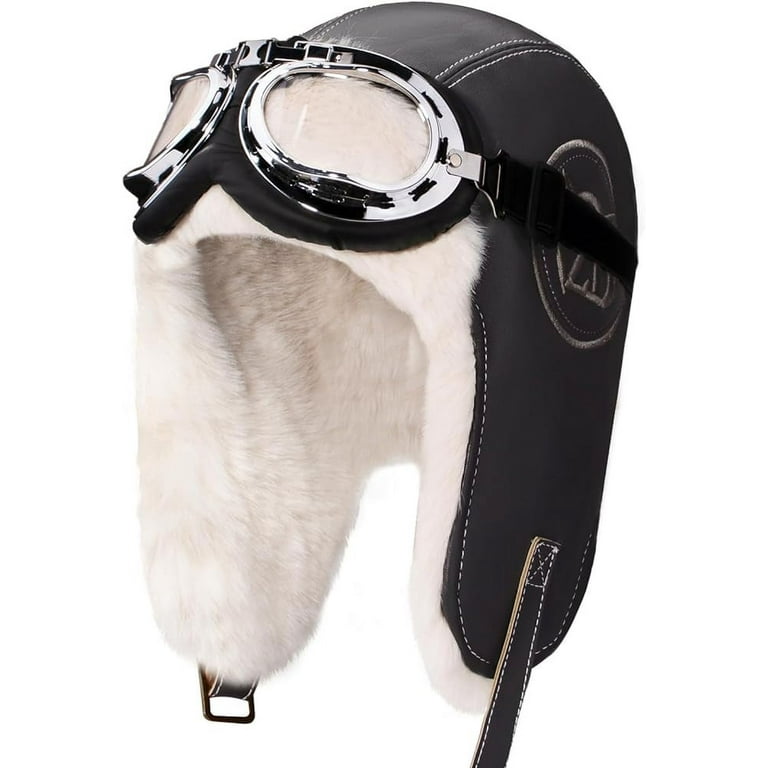This image features a vintage-style aviator's helmet reminiscent of those worn by pilots in WWII bombers or fighter aircraft. The helmet is predominantly black leather, with ear flaps and a fur lining on the inside for warmth, as well as fur trim on the exterior. Notably, there is a detailed stitched design on the side, which is partially obscured by a strap, potentially featuring letters or numbers arranged in a circular pattern. The helmet also includes an unbuckled chin strap extending from one side to the other for secure wear. Resting on the top of the helmet are classic aviator goggles, which have black frames with white detailing and clear plastic lenses. The goggles are positioned across the white fur trim at the top of the helmet and are cushioned with rubber for comfort. The background of the photograph is plain white, emphasizing the helmet as the focal point, suggesting that the image might be intended for product display.